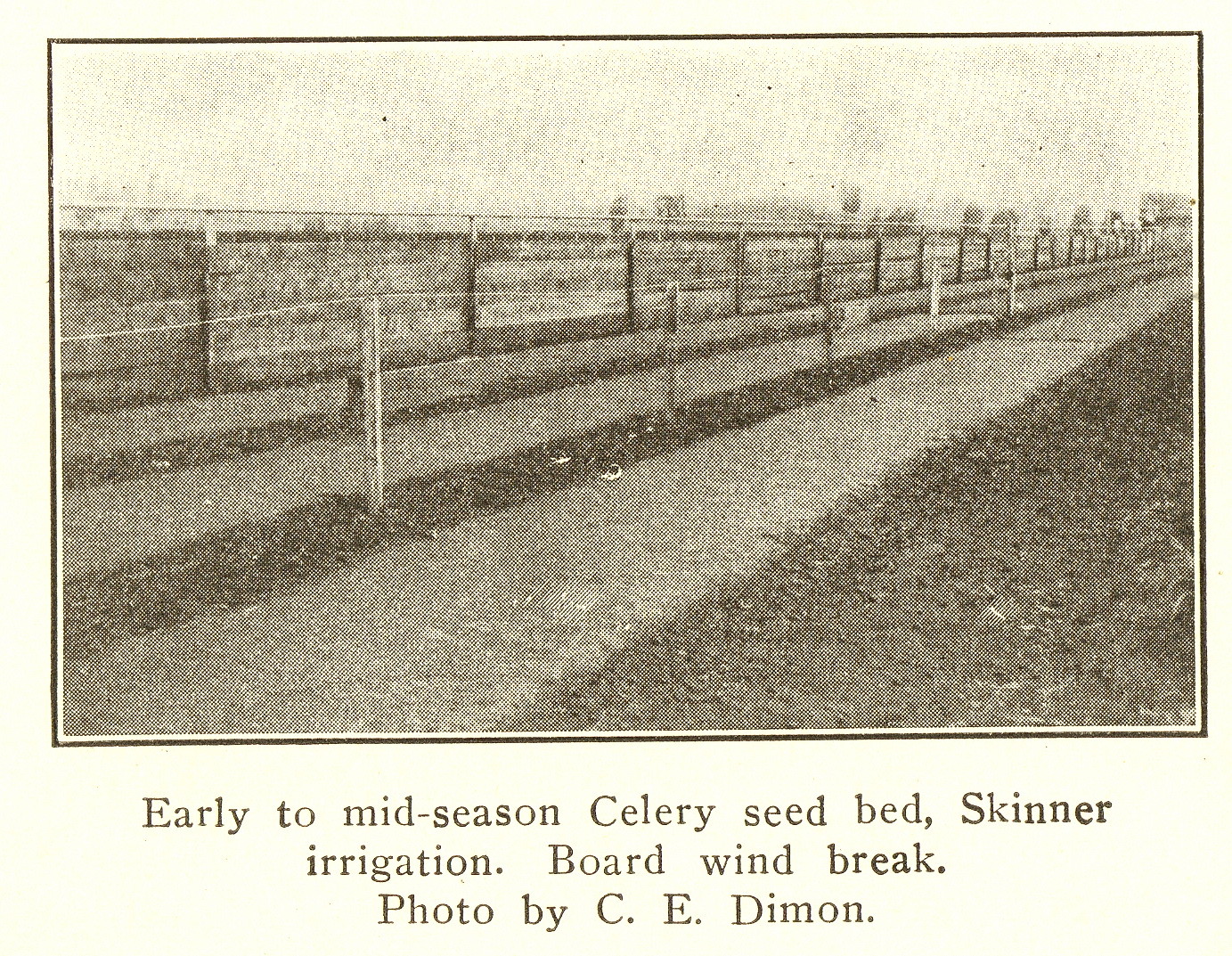This is an old, sepia-toned black-and-white photograph, characterized by its smudgy, blurry, and grainy appearance. The image is framed by a distinct black border, giving it a classic and aged look. It depicts a scene that includes a fence in the foreground and a field in the background, possibly grass or rows of planting. The field appears to have rows of dirt and smoother, lighter-colored areas, with posts sticking out and string or rope connecting them. The photograph is horizontal and rectangular in shape. Below the image, a caption reads: "Early to Mid-Season Celery Seedbed, Skinner Irrigation. Borg Windbreak. Photo by C.E. Dimon." Despite the challenging quality of the photograph, these details provide a glimpse into the early agricultural practices captured by the photographer.